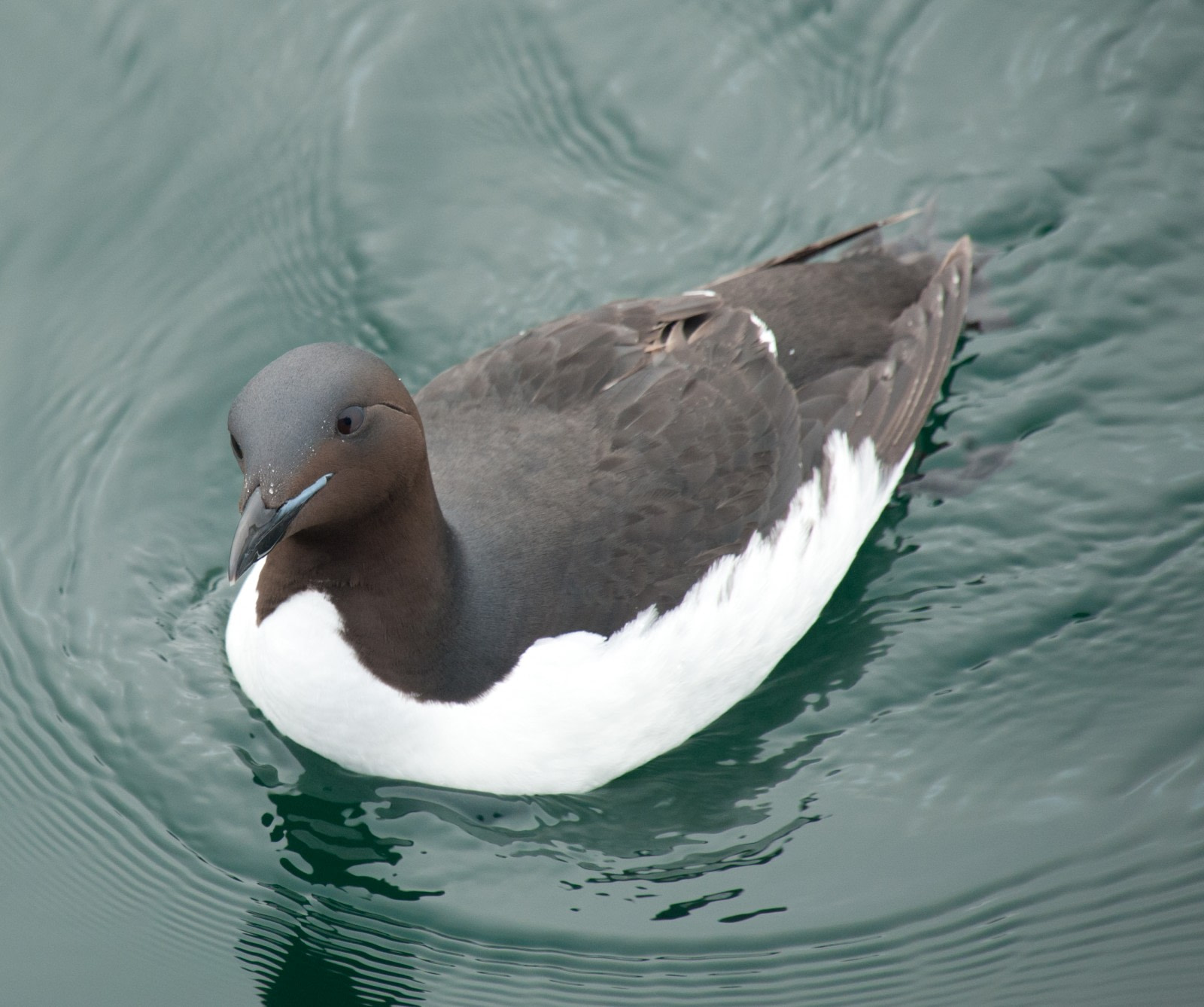This is a full-color, daytime photograph of a duck-like waterfowl with a very unique appearance. The image captures the bird outdoors on greenish water, likely due to algae presence. Swimming on the water's surface, the bird creates a wake behind it and ripples in front. It has a smooth, almost polished head that appears featherless, giving it an uncanny stone-like texture. The bird's dark brown head, neck, and back contrast with its white chest, belly, and sides. The back of its wings, predominantly brown, have a hint of white tips. A delicate hint of blue is visible just behind its beak, where a cheek would be. Its beady black eyes are focused straight ahead, and there's a noticeable wrinkle behind its eye. The square image, with no definitive border, uses natural light to highlight the bird's features against the water backdrop, making the details vivid and lifelike.